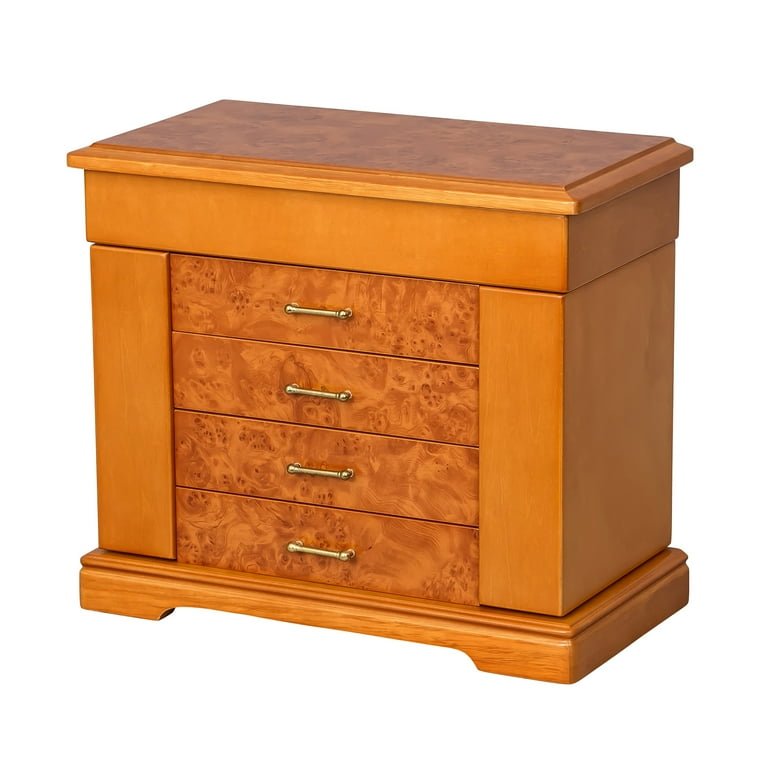This image showcases a sleek, wooden dresser crafted from a light orange-brown wood with a flat top and no legs, presenting a stable base. The dresser features four horizontally aligned drawers in the center, distinguished by their darker, marbled finish which contrasts strikingly with the smooth, lighter exterior. The marbling pattern graces both the drawers and the top surface of the dresser. Each drawer is adorned with a small, silver-toned, flat, arched handle that stretches across its width. The entire piece is captured against a stark white background, emphasizing its detailed finishes and distinctive design elements.